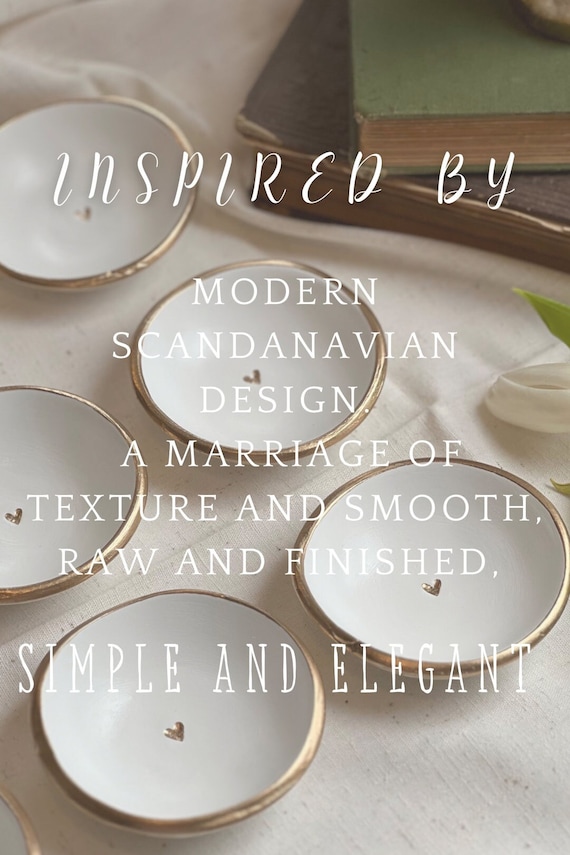The image is a vertically oriented photograph showcasing an elegantly styled table setting. The focal point is five shallow, white bowls, each adorned with a delicate gold rim and a small golden emblem at the center, possibly a decorative painting, though details are minimal. These bowls rest gracefully on a slightly wrinkled white linen tablecloth. Adding a touch of natural elegance, a partially closed white flower, likely a tulip, with visible green leaves, peeks into the frame from the right edge. In the upper right corner, two vintage hardcover books—one brown and one faded green with yellowed pages and worn corners—are stacked atop each other. Overlaying this serene arrangement is white text that reads: "Inspired by modern Scandinavian design, a marriage of texture and smooth, raw and finished, simple and elegant," with the word "inspired" italicized in a handwritten style. This meticulous composition fuses modern design with timeless, rustic elements to create a visually appealing and sophisticated advertisement for dinnerware.